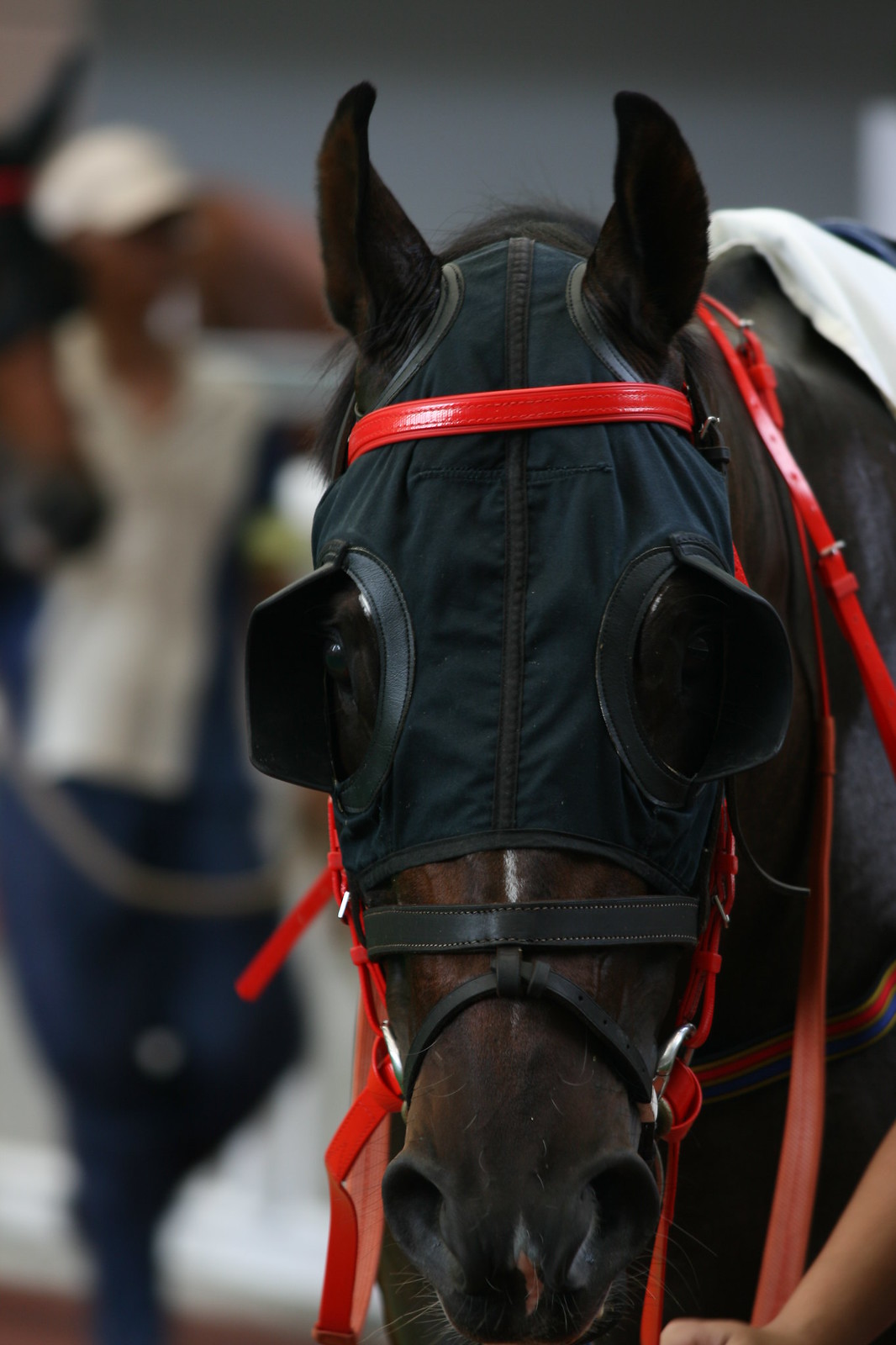This detailed outdoor color photograph features a close-up of a dark brown racehorse's head, adorned with a distinctive black racing mask. The mask covers the top of the horse's head, with oval cutouts for the eyes and ears. The eye holes are lined with black leather trimming, which also includes blinder-like extensions that cup the sides of the eyes to restrict side vision. The horse’s ears point straight up, curving slightly inwards. The mask is secured with multiple straps: a prominent bright red vinyl-looking halter with silver rings and black leather straps that cross the nose and under the chin. The horse also has a silver bit and a partially visible saddle. The blurry background highlights a jockey-like figure dressed in blue and white attire, adding context to the racing scene.